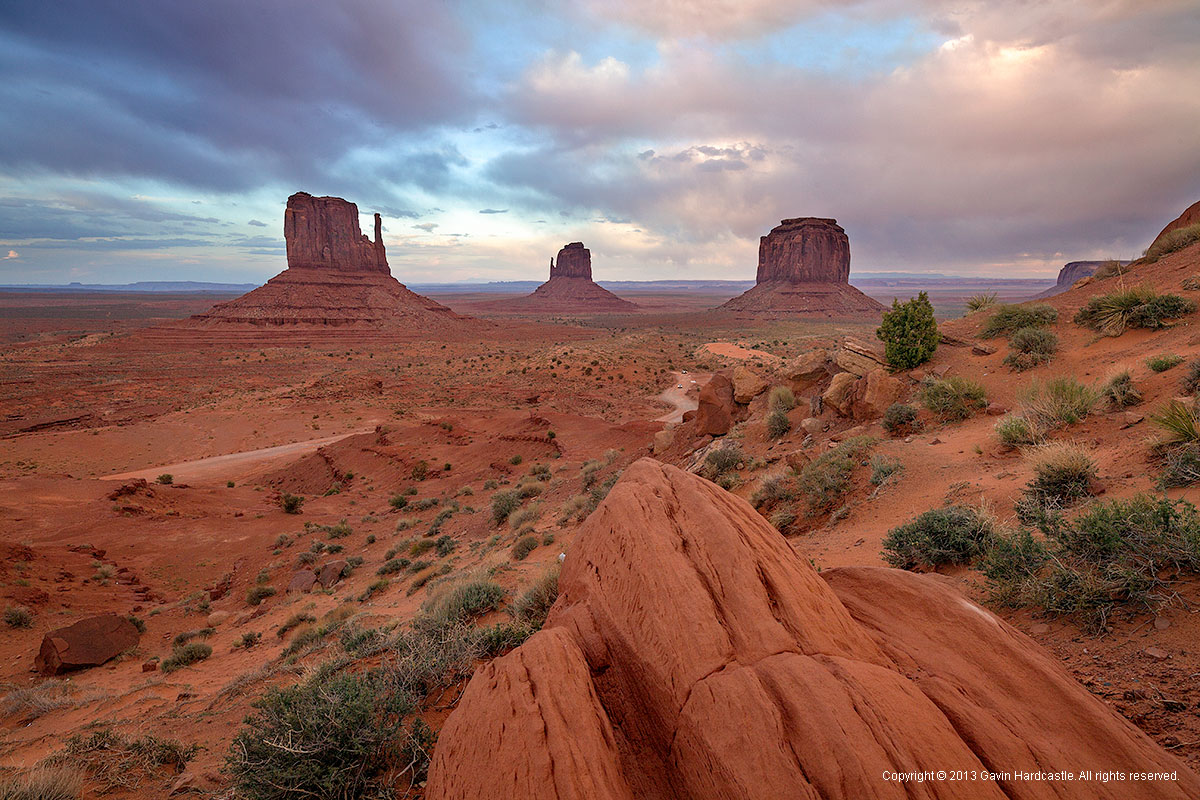The photograph vividly captures a vast desert landscape under a dynamic sky with varying shades of white and gray clouds floating across. Dominating the scene is the iconic, rugged terrain of Arizona, distinguished by its striking orange clay dirt spread across thousands of acres. Prominent orange rock formations punctuate the image; three massive rock structures rise prominently in the distance, with the tallest on the left featuring a broken, thin piece extending from its right end. The middle formation appears smaller due to its farther position, mimicking the shape of the leftmost rock but in reverse. The rightmost structure resembles a large cube capped with a smaller roof-like top. In the foreground, patches of green grass and small ferns contrast the darker brown sand and jagged plateaus. A road subtly traverses the terrain, adding a human touch to this natural expanse. Additionally, a white copyright line reading "Gavin Hardcastle All Rights Reserved" is visible in the bottom right corner of the image, marking the photographer's credit from the year 2013. The overall scene is accentuated by the vibrant blue sky, further enhancing the natural red and green hues below.